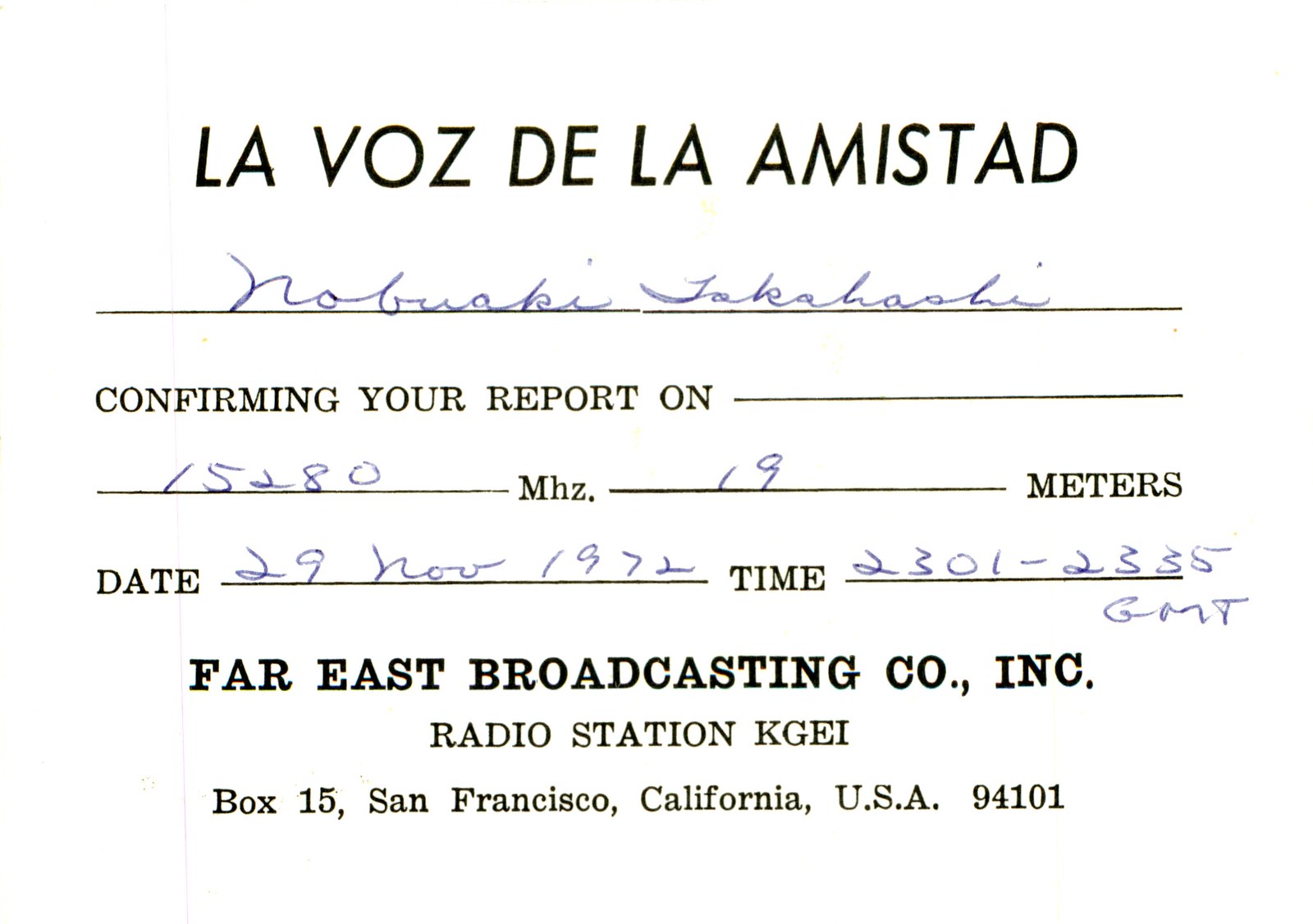This black and white scanned image is a vintage, landscape-oriented postcard form. The top of the form features the headline "LA VOZ DE LA AMISTAD" in bold, black capital letters against a white background. Below this is a horizontal line, upon which is written "Nobuaki Takahashi" in elegant cursive handwriting. Further down, the form reads in print, "Confirming your report on," followed by blank spaces filled with the technical details "15280 MHz" and "19 meters." The date "29th November 1972" and the time "2301-2335 GMT" are also hand-filled in blue pen. At the bottom of the form, the printed text reads, "Far East Broadcasting Company, Inc., Radio Station KGEI, Box 15, San Francisco, California, USA 94101."